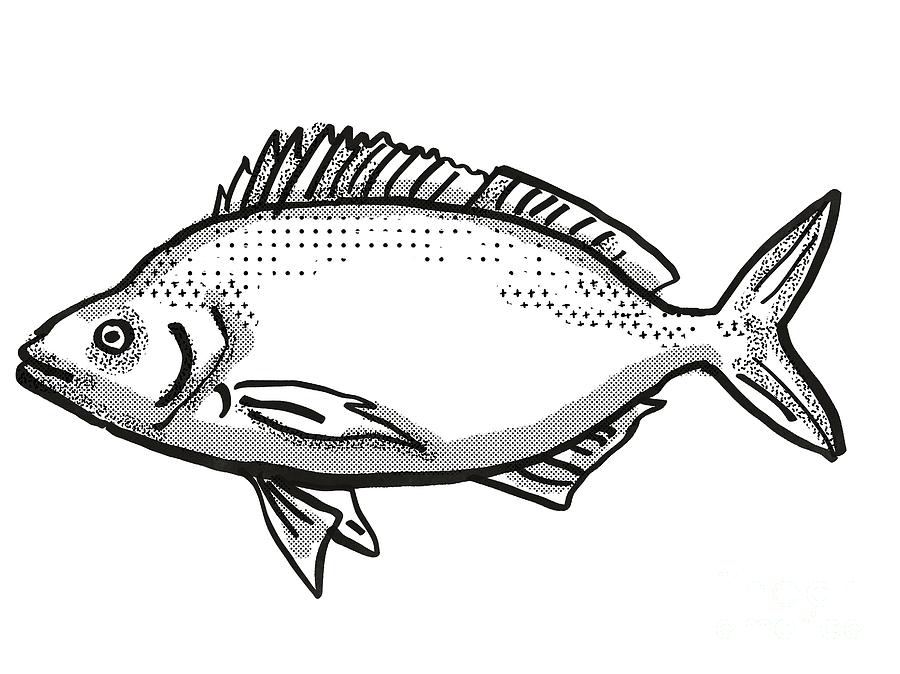This black and white illustration showcases a fish in a side profile, with its head facing left and tail to the right, set against a plain white background. The fish is portrayed with a pointy mouth and a subtle dimple on its head. Detailed with varying line widths that appear to be drawn with a marker, the artwork emphasizes the texture and form of the fish. Its body features a series of small dots and x marks from head to tail, contributing to the shading and texture, with more concentrated dot patterns along the outline creating a gray gradient effect.

The fish's anatomy is distinctly illustrated with prominent gills, a jagged long top fin that becomes flatter and runs parallel to its body towards the tail, and three fins at the bottom—one near the head, one near the belly, and another towards the tail. The tail fin itself is dotted on both sides. The overall shading and texture use a combination of tight dot patterns and more spaced-out dots, giving the fish a dynamic, almost halftone-like appearance, while parts of the shading resemble black and white noise or static. The fins, eyes, and mouth are rendered with clear attention to detail, completing the lifelike yet artistic representation of the fish.